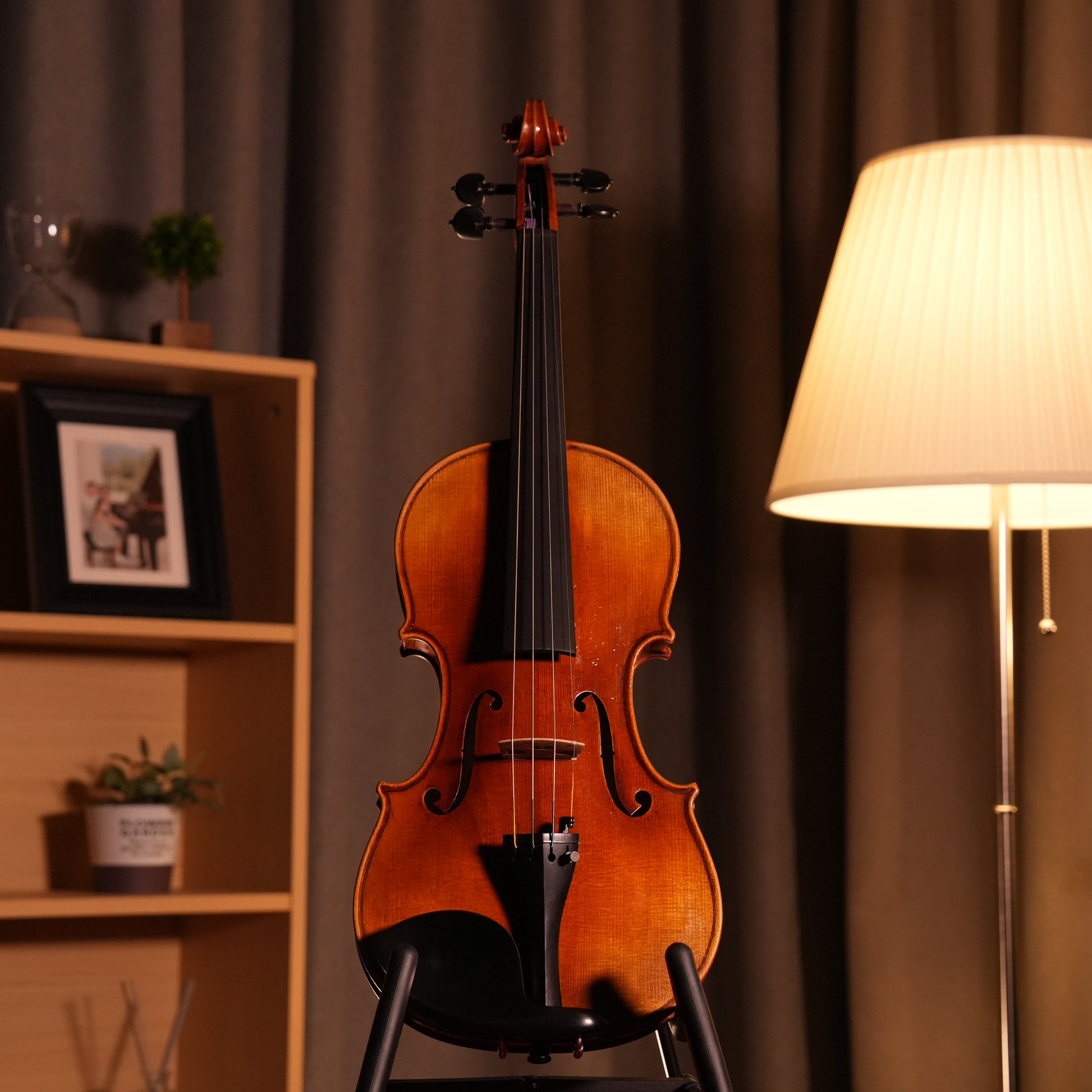This color photograph, shaped as a square, prominently features a vertically oriented violin perched on a black stand at the central part of the image. The violin itself is a striking cherry wood color with dark ebony accents on the neck and chin rest, complemented by light-colored strings and four tuning pegs at the base. To the right of the violin stands a lit floor lamp with a pleated white shade and a pull chain, casting a warm glow across the scene. The backdrop is completely covered by large brown drapes, creating a rich and somewhat cozy ambiance. On the left side of the violin, a bookcase is visible with a variety of items: a potted plant occupies the middle shelf, stemware glasses are on the lower shelf, and the top shelf showcases a framed photograph along with miniature topiary knickknacks. The detailed composition and lighting of the photograph bring a harmonious balance between the richly textured violin and its surrounding elements.